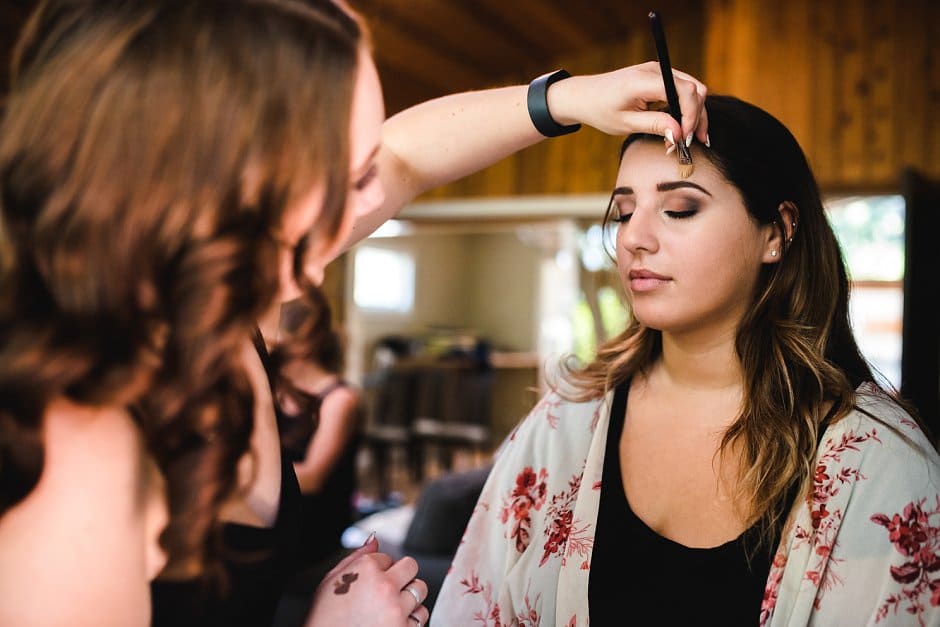The image features a young woman seated in a chair, having her makeup expertly applied by another woman standing beside her. The makeup artist, who has dark brown hair with wavy, curly ends and is wearing a black wristband, uses a black-handled brush with light brown bristles to work on the area above the young woman’s left eyebrow. The seated woman has sleek, dark brown hair with blonde highlights towards the ends that cascade below her chest. She is dressed in a black tank top partially covered by a sheer white camisole with a red floral pattern. Her smoky eye makeup and polished pink-hued lips enhance her youthful face, and she has earrings in her ears. The setting appears to be a wooden building, with dark wood visible on the ceiling and blurred black chairs in the background, along with another indistinct figure. The overall ambiance, softened by natural light from a window, creates an intimate and focused moment of beauty application.